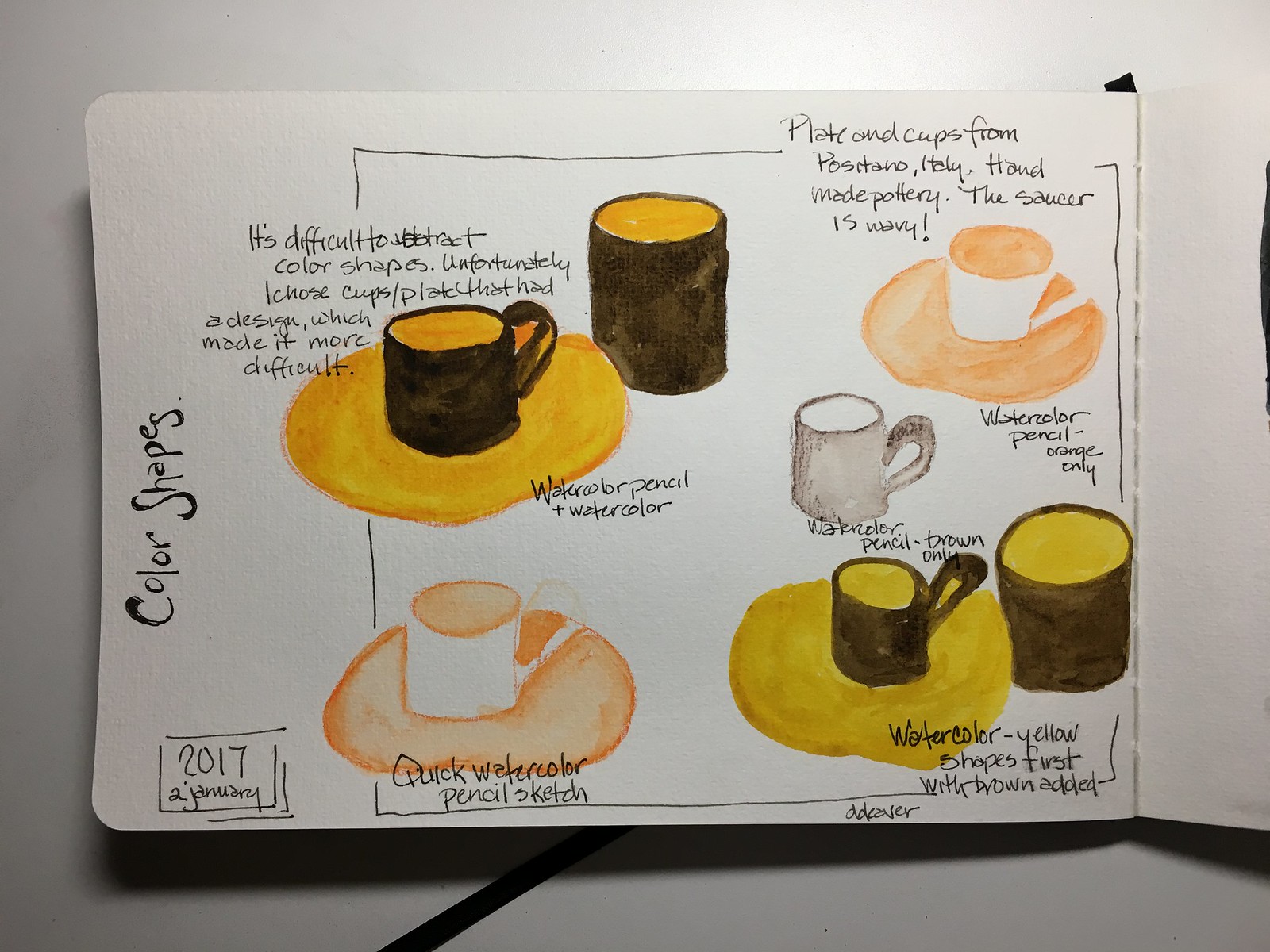This photograph captures a detailed and artistic drawing in a notebook against a white backdrop. The notebook page itself is white, providing a clear canvas for the artwork. A black ribbon, likely serving as a bookmark, dangles from beneath the notebook, adding a contrasting touch.

The drawing prominently features an array of coffee cups and saucers, depicted in various shades and hues. On the left side of the page, the words "Color Shapes" are written in black. A small rectangular box beneath this text contains the date "2017 to January."

Several specific notes about the drawing are scattered around the page:
- "Watercolor pencil orange only" and "Watercolor pencil brown only" detail the media used for one of the depicted cups.
- "Watercolor yellow shapes first with brown added" describes the technique used for coloring some of the cups.
- "Quick watercolor pencil sketch" references a white cup with orange liquid and an orange shadow underneath.
- Another note mentions the challenge of using watercolors to abstract color shapes, particularly because the chosen cups and plates had intricate designs.

The artwork includes a yellow-colored plate and two black cups, each with yellow interiors. Further text reveals that these are plates and cups from Pastino, Italy, handmade from pottery, and the saucer features a distinctive wavy design. This descriptive annotation highlights the artist's attention to detail and the intricate process involved in creating the drawing.